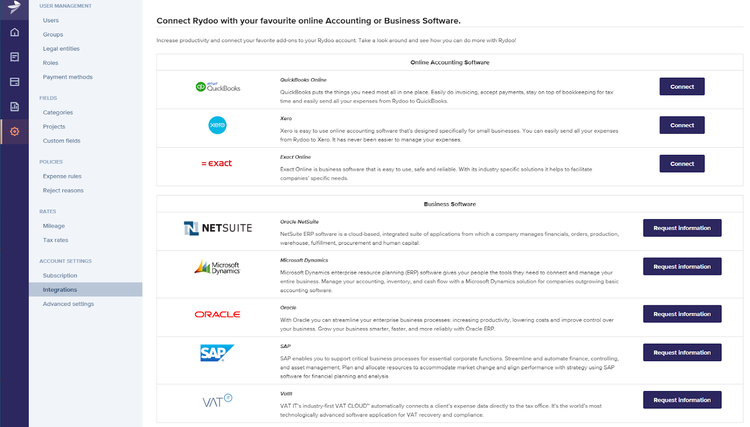This image showcases a menu page from an online user guide or manual, featuring a structured layout with distinct sections for easy navigation. On the left side, there is a vertical navigation pane designed in a purple hue, populated with various icons occupying the top one-third of the panel. At the top is the brand icon, resembling a dove in flight towards the right. Beneath it, from top to bottom, are icons representing different functions: a home button, a document-like icon indicating text, an envelope icon suggesting messages, a chart icon for reports, and a settings wheel, which is highlighted in orange to indicate it is currently selected.

Adjacent to this panel, a second vertical navigation box lists text-based options under a “User Management” title. These options include: Users, Groups, Legal Entities, Roles, Payment Methods, Fields, Categories, Projects, Custom Fields, Policies, Expense Rules, Reject Reasons, Rates, Mileage, Tax Rates, Account Settings, and Subscription. Below this list, “Integrations” is highlighted in dark gray, signifying its active status, followed by the “Advanced Settings” option.

The remaining 80% of the image on the right side displays the contents of the selected page, which focuses on integrating with various accounting and business software. The page header reads: “Connect Raidu with your favorite online accounting or business software.” Below this is a table featuring a list of software programs segmented into two categories: "Online Accounting Software" and "Business Software."

Each software is represented by three columns: a logo in the leftmost column, the software name in the middle column, and a button in the rightmost column which is purple with white text. Accounting software brands shown include QuickBooks, Xero, MYOB, and Exact, each accompanied by a "Connect" button. Business software brands listed are NetSuite, Microsoft Dynamics, Oracle, SAP, and VAT, each having a "Request Info" button instead. The table is divided by a heading row labeling the top section "Online Accounting Software" and the bottom section "Business Software."

This clean, detailed layout enhances user experience by clearly differentiating between various navigation options and seamlessly displaying integration possibilities with popular accounting and business software.